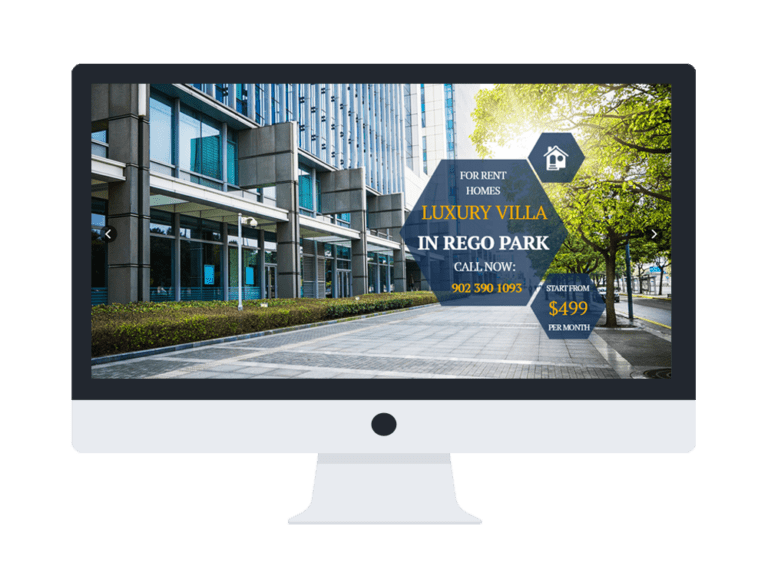The image showcases a computer-generated white flat-screen monitor mounted on a sleek pedestal, set against an entirely white background. The monitor's design is minimalist, featuring a thin black frame around the screen and a small black button at the bottom center. Displayed on the screen is a vibrant photograph of a town street lined with modern high-rise buildings. Among the towering structures, one building on the left prominently displays a sign that reads, "For Rent: Luxury Villa in Rego Park. Call Now 902-390-1093. Starting from $4.99 per month." The text on the sign is in alternating white and orange fonts.

The depicted scene includes green trees and manicured bushes that add a touch of nature to the urban landscape. The buildings in the image, especially one with a glass facade, have a bluish tint, emitting a modern, sophisticated vibe. Additionally, there is a brick walkway with grayish tones, leading through the area. Sunlight filters through, casting subtle shadows and enhancing the realism of the scene.

Overlaying the photograph is a semi-transparent honeycomb pattern composed of hexagons, allowing glimpses of the image underneath. Despite the intricate details, the entire visual presentation has an artificial, computer-generated aesthetic. The white background of the monitor blends seamlessly with the white background of the scene, contributing to the overall synthetic appearance.